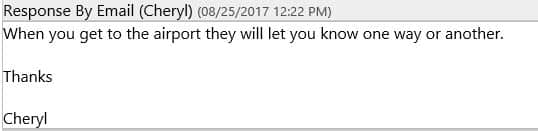Response by email from Sheryl A on August 25, 2017, at 12:22 p.m.: "When you get to the airport, they will let you know one way or another. Thanks, Sheryl." Additionally, she notes, "Once you're on your way back, there's a gray line, and your brother will let you know one way or another. Thanks, Sheryl."

In the background, the image is somewhat unclear with a static effect.